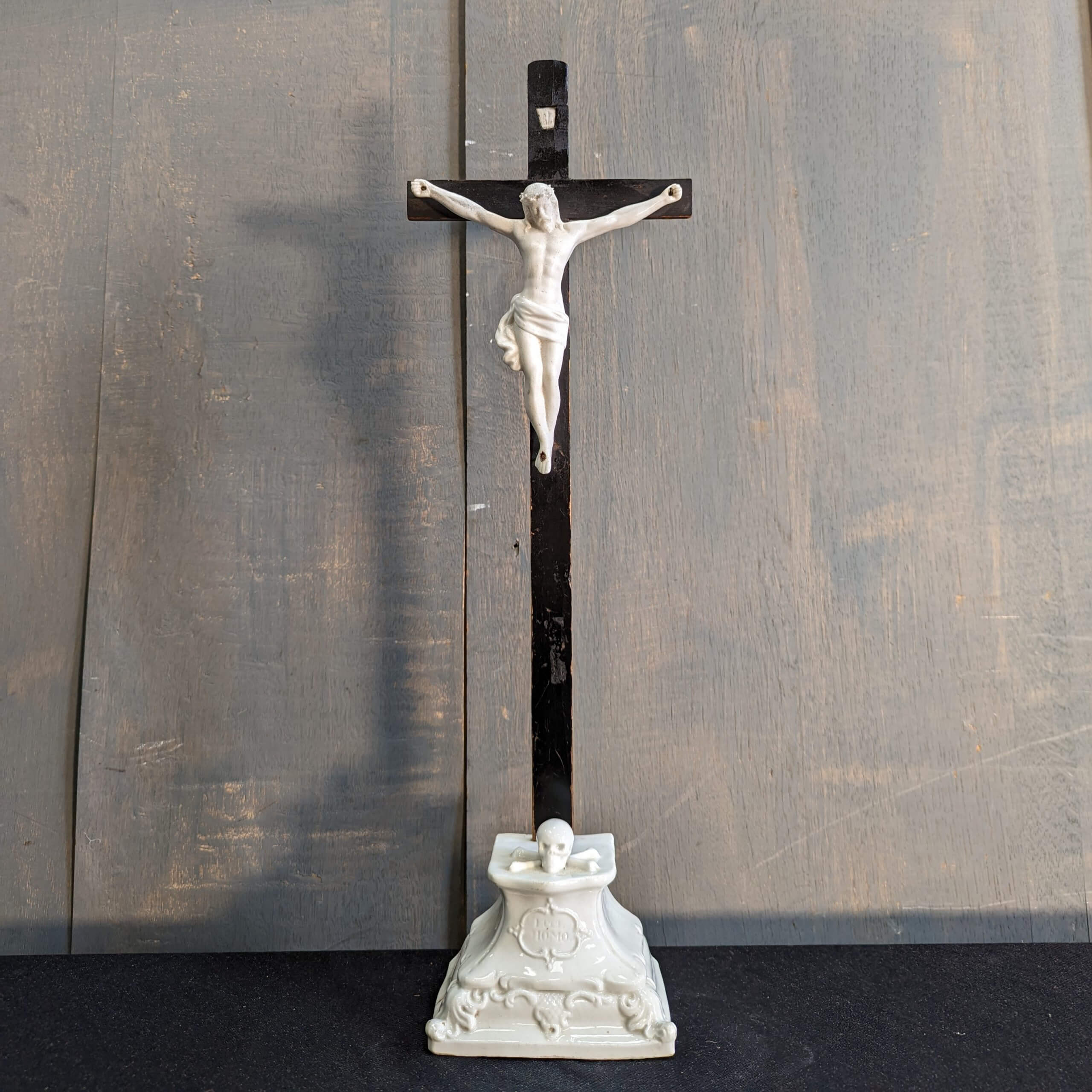The image depicts a detailed and somewhat rustic crucifix scene. At the forefront, a wooden cross hosts a cream-white, ceramic figure of Jesus Christ. Jesus is depicted in the traditional crucifixion posture with nails in his hands and a cloth draped around his waist, complemented by his beard and solemn expression. Above his head is a small, white piece of paper with a smiley face on it. The cross stands against a backdrop of worn wooden panels that appear to have been haphazardly painted gray, allowing the natural wood texture to peek through. 

At the base of the cross, there's an ornate, white stand that features delicate, regal patterns etched into the ceramic. Prominently displayed on this stand is a small skull and crossbones, approximately one inch high, sitting next to the bottom of the cross. The entire structure rests on a dark, possibly black, floor which contrasts starkly against the lighter hues of the cross and figure. The intricate details of this piece, including the hand-etched designs and meticulous portrayal of Jesus, give it a captivating, almost ceremonial appearance, reminiscent of traditional Catholic iconography.